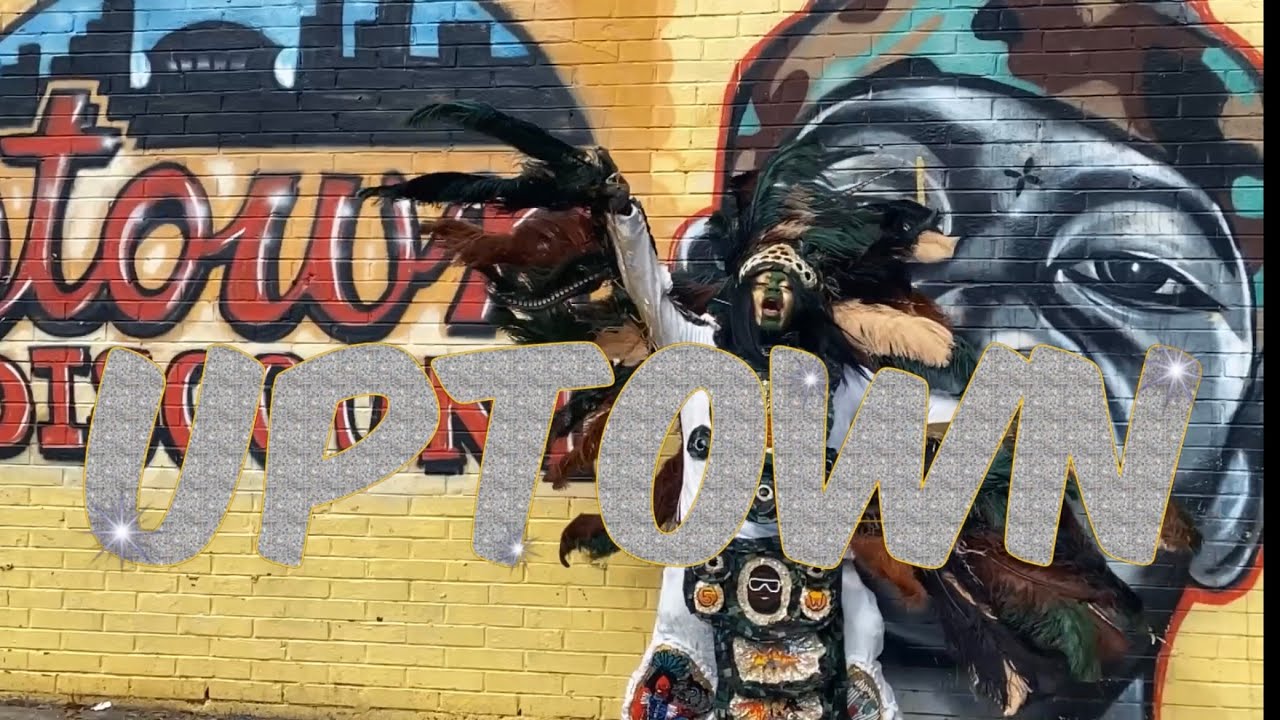This detailed, up-close photograph showcases a vibrant mural on the yellow-painted brick side of a building. Central to the artwork is the word "Uptown" in gray with a yellow outline, positioned slightly below the midline. Behind this text, a multifaceted mural emerges, featuring a culturally diverse figure. This man, dressed in a white outfit adorned with multicolored tattoos, has vibrant black hair and a headdress with black feathers. His face is marked by striking yellow paint. To his right stands a young black male adorned with a camo-patterned headband in shades of blue, brown, and black, with a distinct black cross tattoo on his forehead. In the top left corner, there's a partial blue sky and black high-rise buildings, framed in a half-circle mural segment with red cursive letters, partially visible as "T-O-W", trimmed in black. The complexity and detailed elements of the mural blend graffiti art with professionally painted storytelling, highlighting an urban cultural narrative.